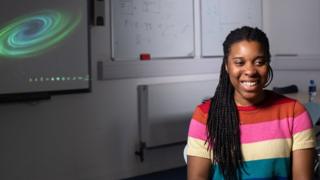In this image, a cheerful woman with dark skin and black hair is captured smiling at the right side. She is wearing a short-sleeved top featuring a vibrant array of colors: a red band at the top with a red collar, followed by horizontal stripes in brown, pink, yellow, and green. Behind her, the off-white wall serves as a subtle backdrop. On the left side of the image, a grey screen displays a swirling green pattern, which resembles a wormhole or black hole, along with some white or greenish text that's somewhat difficult to read. Additionally, there are whiteboards behind her, marked with writing in possibly dark blue ink and featuring a small red square at the base. A square object is also mounted on the wall. Her radiant smile and the colorful background create a lively and engaging scene.